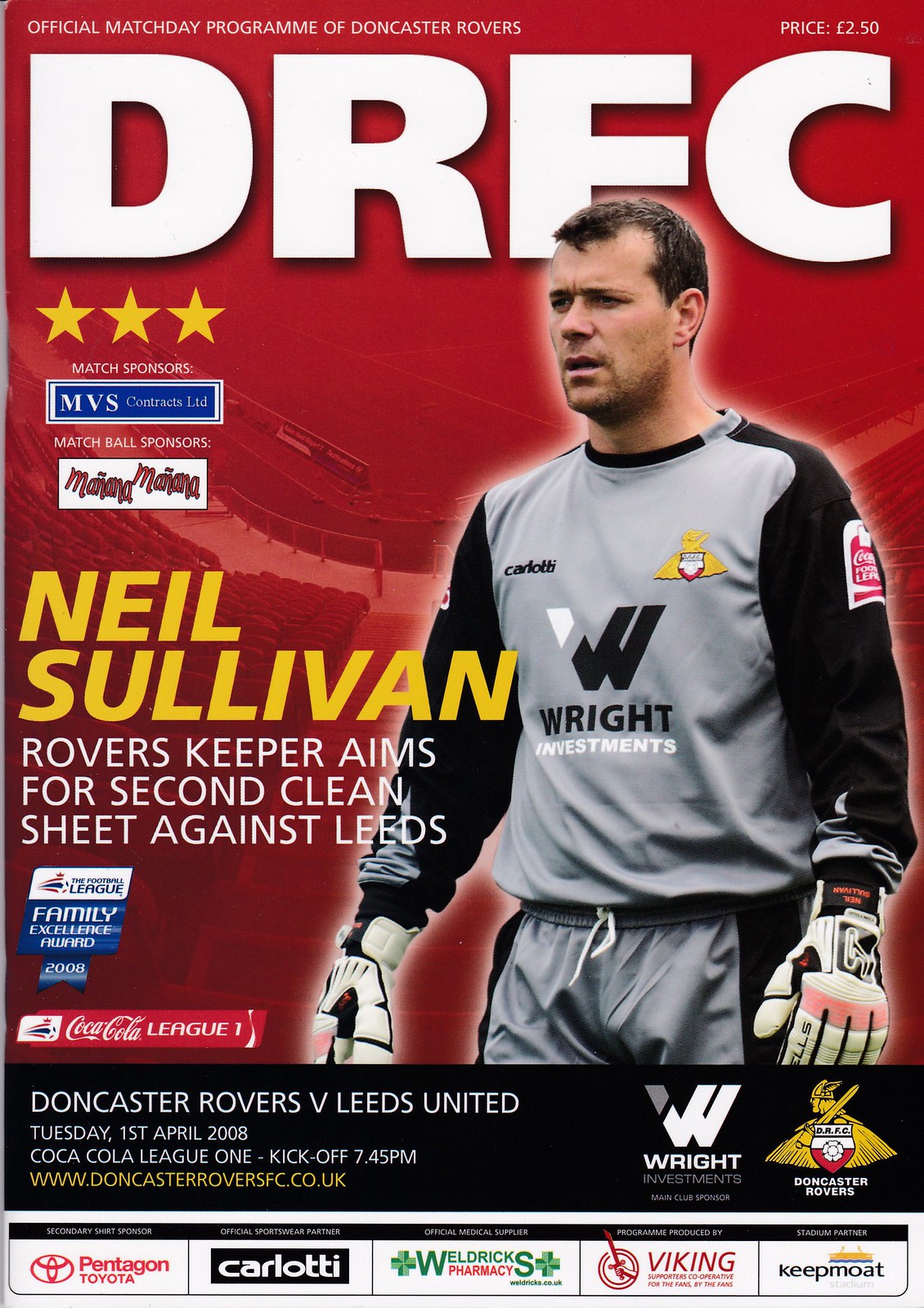This is a magazine cover for an official match day program of Doncaster Rovers. At the top, in white block letters, it says "DRFC." Below, it lists the price as $2.50. The main image features a man on the left, identified as Neil Sullivan, wearing a gray shirt with black sleeves. The word "Wright Investments" with a black W is prominently displayed on his shirt. He's sporting white mechanics gloves and has a serious expression with his mouth slightly open, dark hair, and a hint of a beard and mustache. The background is red with the magazine title in white letters at the top.

To the left, there are three stars followed by "Match Sponsors: MVS" and "Match Ball Sponsors," with an indistinct logo beneath. In yellow letters, it reads "Neil Sullivan," followed in white letters by "Rovers keeper aims for second clean sheet against Leeds." Various logos, including Coca-Cola, are scattered underneath with accompanying text: "Doncaster Rovers vs. Leeds United." Additional sponsor logos at the bottom include Pentagon, Toyota, Carlotti, Weldrick Pharmacy, Viking, and Keepmoat. The magazine also notes the date, Tuesday, 1st April 2008, Coca-Cola League One, and the kickoff time at 7:45 p.m., along with the website information.